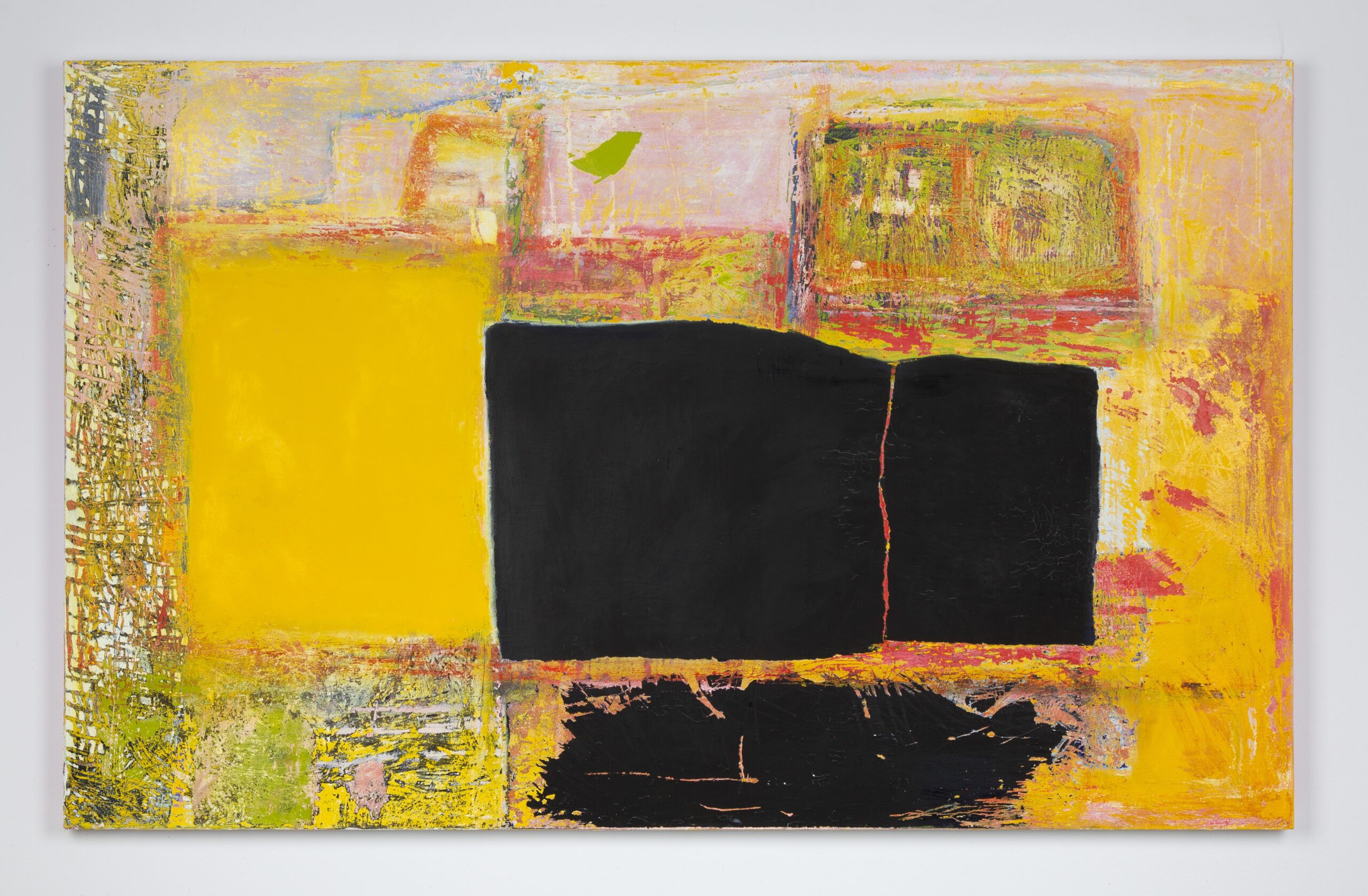In this image, we see an abstract painting with a primarily white border, giving it a frameless appearance that blends into the wall. The artwork is centered around geometric and cubist elements, dominated by various squares and rectangles in a vivid palette. Yellow hues with varying textures fill much of the canvas, accompanied by prominent black squares in the middle with jagged edges, suggesting a dynamic, almost chaotic feel. Towards the bottom left, there is a blend of green and pink, appearing as if drawn with markers in a scribbled fashion. Light pink and a lime green with reddish scribbles are present at the top, contrasting with the smoother, brighter yellows on the left and the messier textured yellows to the right. Overall, the piece exudes a modern, contemporary vibe with its interplay of bold colors and abstract forms.